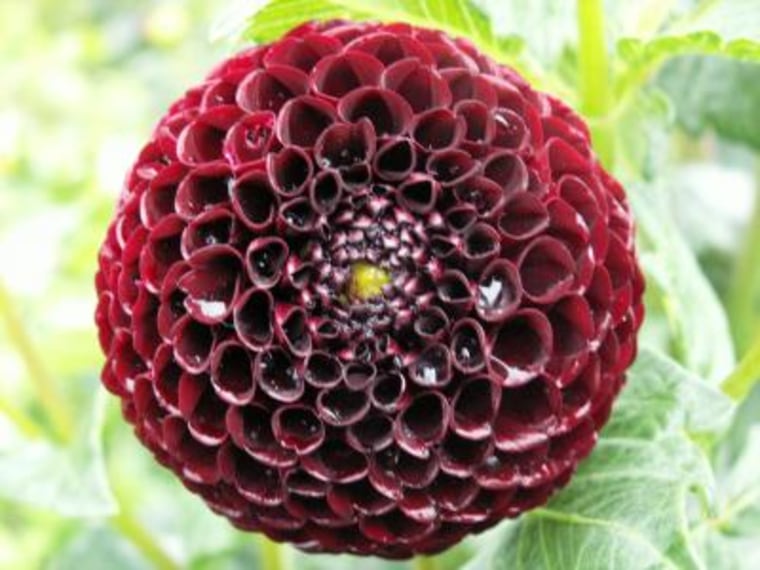This is a square photograph capturing a striking close-up of a flower, likely a Dahlia. The flower, occupying about 75% of the frame, is a rich maroon color with a subtle gradient, appearing darker toward the center and lighter at the edges. The petals are tightly curled into tubular shapes, giving the flower a textured, multi-dimensional appearance reminiscent of small cornucopias or craters. At the heart of the flower lies a smooth, yellow dot, evocative of rounded beeswax or a mirrored disco ball. The overall shape of the flower is circular, composed of numerous smaller circular formations.

The background is softly blurred, accentuating the flower's detailed structure, while a hint of light green foliage frames the composition. Although this foliage resembles cabbage leaves, it remains ambiguous whether the dahlia is directly attached to them. Delicate water droplets are visible on the petals, suggesting either morning dew or recent rainfall, and a light dusting of white powder hints at the possibility of frost or snow, further adding to the image's intricate beauty. The excellent natural lighting illuminates the flower, emphasizing its vibrant hues and fine details.